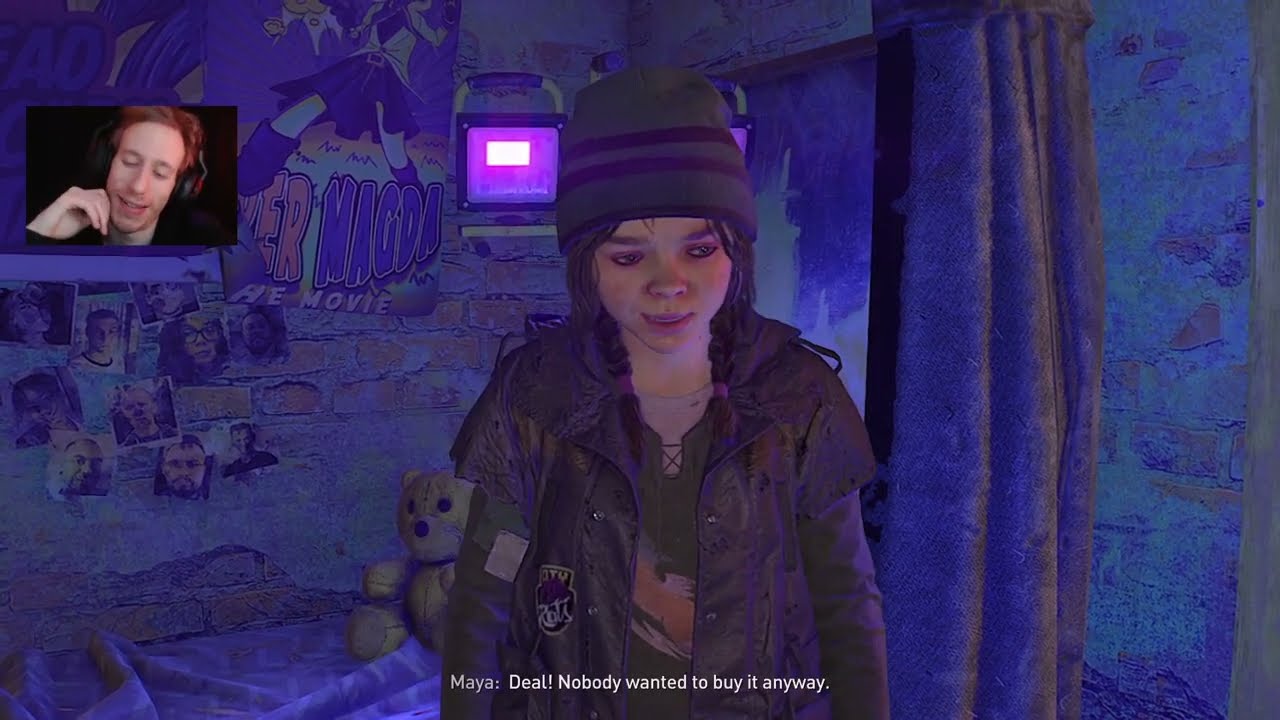The image appears to be a snapshot from a video game stream, possibly on Twitch. In the upper left-hand corner is a small black rectangle showing a red-haired man wearing a headset, who seems to be the streamer, likely describing the events in the game. The main focus of the image is a young girl positioned in the center. She is wearing a purple-striped stocking cap and a grungy, dark jacket layered over a green shirt with some writing on it. Her image is cut off at the waist by white text that reads, "Maya: Deal, nobody wanted to buy it anyway."

The girl is looking slightly downward and to the right. To her left (on the image's right) is a bed with a stuffed teddy bear on it. Behind her, there is a wall decorated with various photographs and drawings, including some that appear to be of people and anime characters. There's a curtain and a window visible in the background, as well as a lit TV monitor on a shelf. The overall background color of the scene is shaded in dark blue and purple hues, suggesting that the setting might be a dimly lit room, perhaps a cellar. The detailed setting and character, along with the displayed text, emphasize that this scene is part of a narrative within a video game.